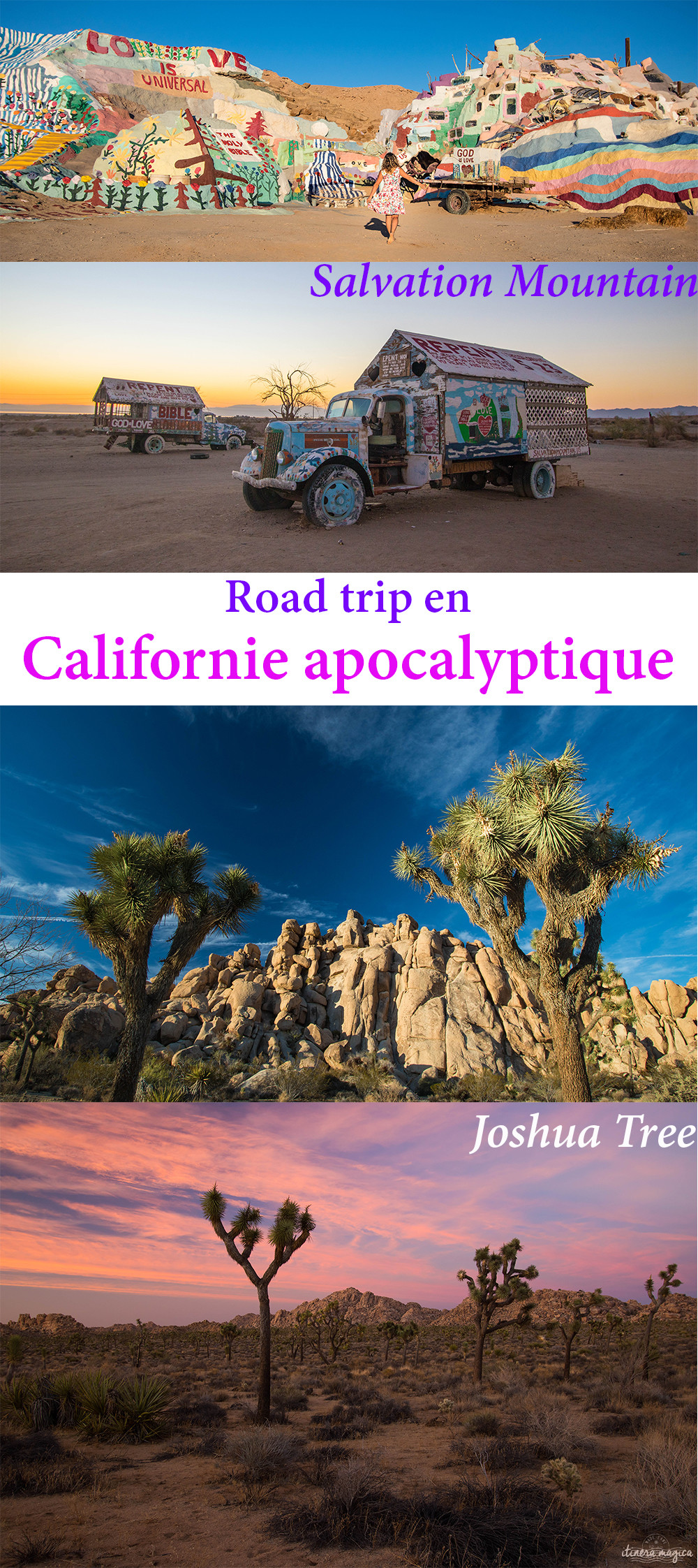This image collage captures the eclectic and vibrant essence of travel through California. The top section prominently features two striking photos of Salvation Mountain, an art installation in the desert known for its colorful murals and religious messages. The first of these photos showcases a painted hillside with bright hues and inscriptions like "Love is Universal" and "God is Love." In front of the hill sits a woman in a floral dress, gazing at the art. The second Salvation Mountain photo, taken at sunset, depicts a whimsically painted truck with a small house in its bed, a nod to the artist’s former residence. 

Separating the two sections of the collage is a bold text reading "Road Trip" and underneath, "California Apocalyptique" in purple letters.

The bottom section of the image highlights two photos of Joshua Tree National Park. The top photo is a breathtaking daylight shot of spiky-leaved Joshua Trees set against a backdrop of cliffs and a bright blue sky. Below this, the final image captures the trees at dusk with a stunning purple-pink sky, showcasing the serene beauty of the desert landscape. Together, these images create a vivid portrayal of a whimsical, apocalyptic road trip through California’s most iconic desert locations.